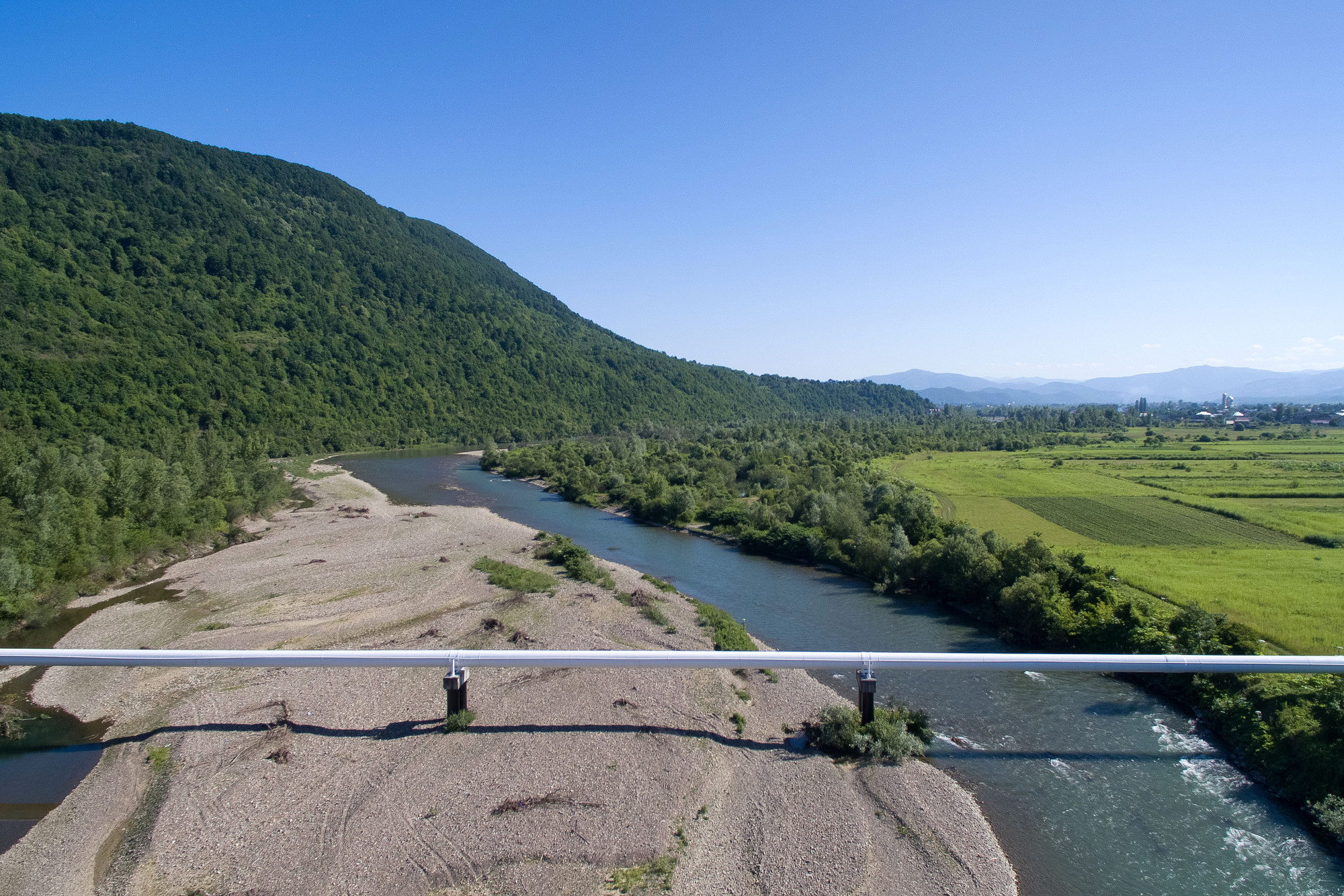This outdoor photograph captures a sunlit scenic vista featuring a countryside landscape. In the background, tall, majestic mountains stretch across the horizon, with a bright blue sky overhead. Closer to the photographer and framing the scene on the left, a verdant mountain covered in lush greenery dominates the view. A significant white pipeline, supported by visible buttresses, bisects the image, running horizontally from the left edge across a sandy area and a winding river or large stream that curves through the middle of the picture. On the right side of the river, which bends up and to the left before disappearing behind a grove of trees, green fields stretch out, accompanied by more brush and rolling hills further in the distance. In the far right of the image, below the distant mountains, a cluster of buildings suggests the presence of a small city or town, further contributing to the serene and varied landscape. The purpose and contents of the pipeline remain unknown, adding an element of mystery to this picturesque countryside scene.